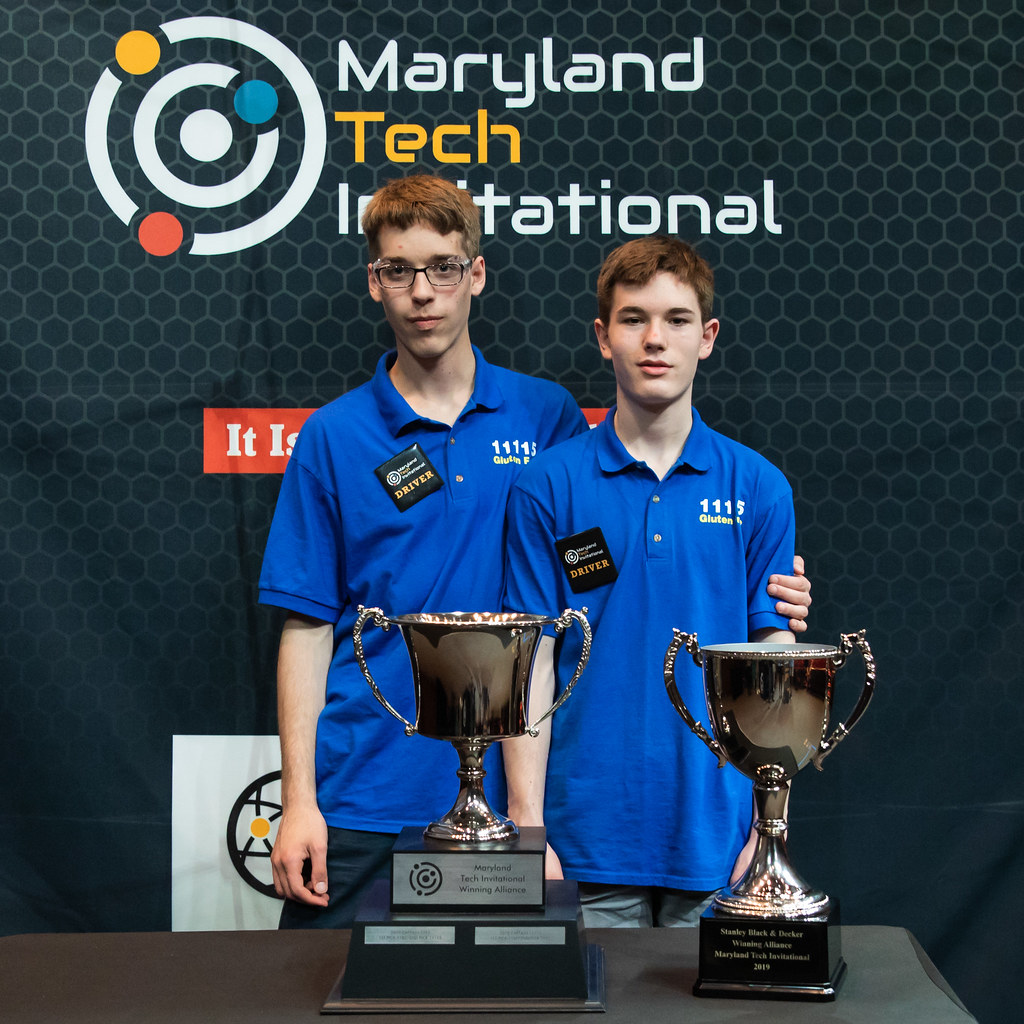In this vibrant color photograph, two teenage boys stand prominently in the foreground, proudly displaying their achievements. Both boys, who have red hair and are Caucasian, are dressed in matching blue polo shirts featuring the number "1-1-S" on the left chest area and a black badge labeled "DRIVER" in orange. The boy on the left, who is slightly taller and wears glasses, has his arm affectionately draped over the shoulder of the boy on the right. 

Directly in front of them on a gray table are two impressive silver trophies, each mounted on a black base, although the detailed inscriptions on them remain unreadable. 

The backdrop is a striking black and gray hexagonal design, primarily decorated with text. Above their heads, the words "Maryland Tech Invitational" are prominently displayed; "Maryland" and "International" are rendered in white text, while "Tech" is highlighted in yellow. To the left of this text is a distinctive bullseye symbol comprised of concentric white circles interspersed with blue, yellow, and red dots. This overall composition underscores a moment of pride and recognition at the Maryland Tech Invitational event.